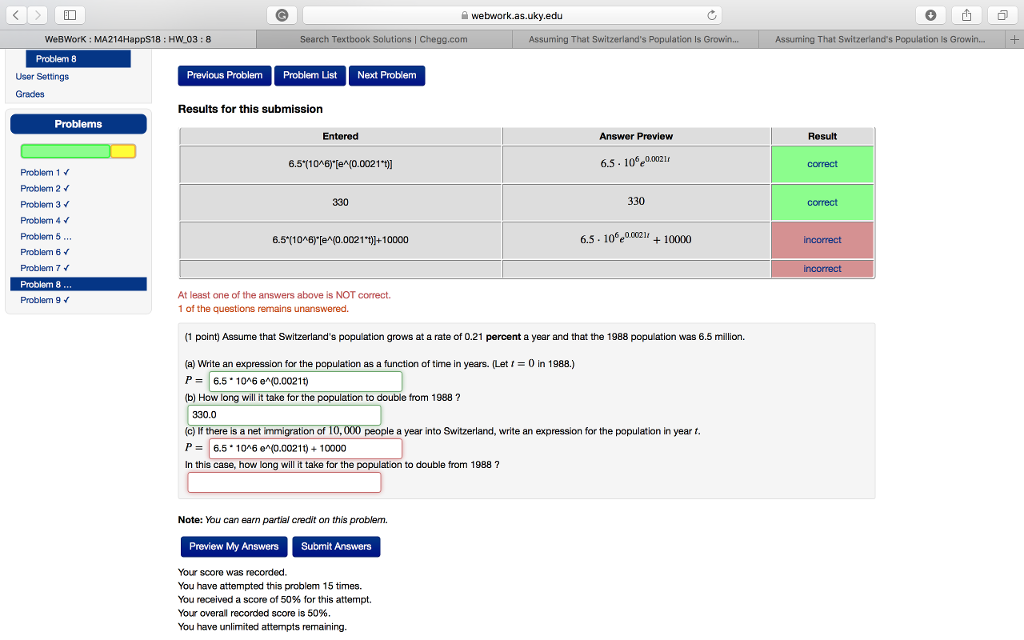This image is a screenshot taken from a cell phone displaying a web-based homework interface, specifically from WebWork, as indicated by the URL "webwork.as.uky.edu" at the top. The interface features a navigation bar that includes clickable links labeled "Previous Problem," "Problem List," and "Next Problem." The user is currently viewing Problem 8 out of a series of nine problems.

The main section of the screenshot shows the problem-solving interface, where users can input their answers. Below each input field, there is a detailed review of the submitted answers. The interface shows both the student's submitted answers and a preview of those answers, segregated by correctness. The feedback is color-coded: correct answers are marked in green, while incorrect answers are marked in red. In this particular submission, the top two answers are correct, and the bottom two are incorrect. Furthermore, one question remains unanswered.

A notification at the bottom of the problem feedback states: "At least one of the answers above is not correct. One of the questions remains unanswered." This is followed by buttons labeled "Preview My Answers" and "Submit Answers." The student's performance on this attempt is also summarized, indicating that they received a score of 50% for this session. Their overall record score is also 50%, with a note that unlimited attempts are allowed.